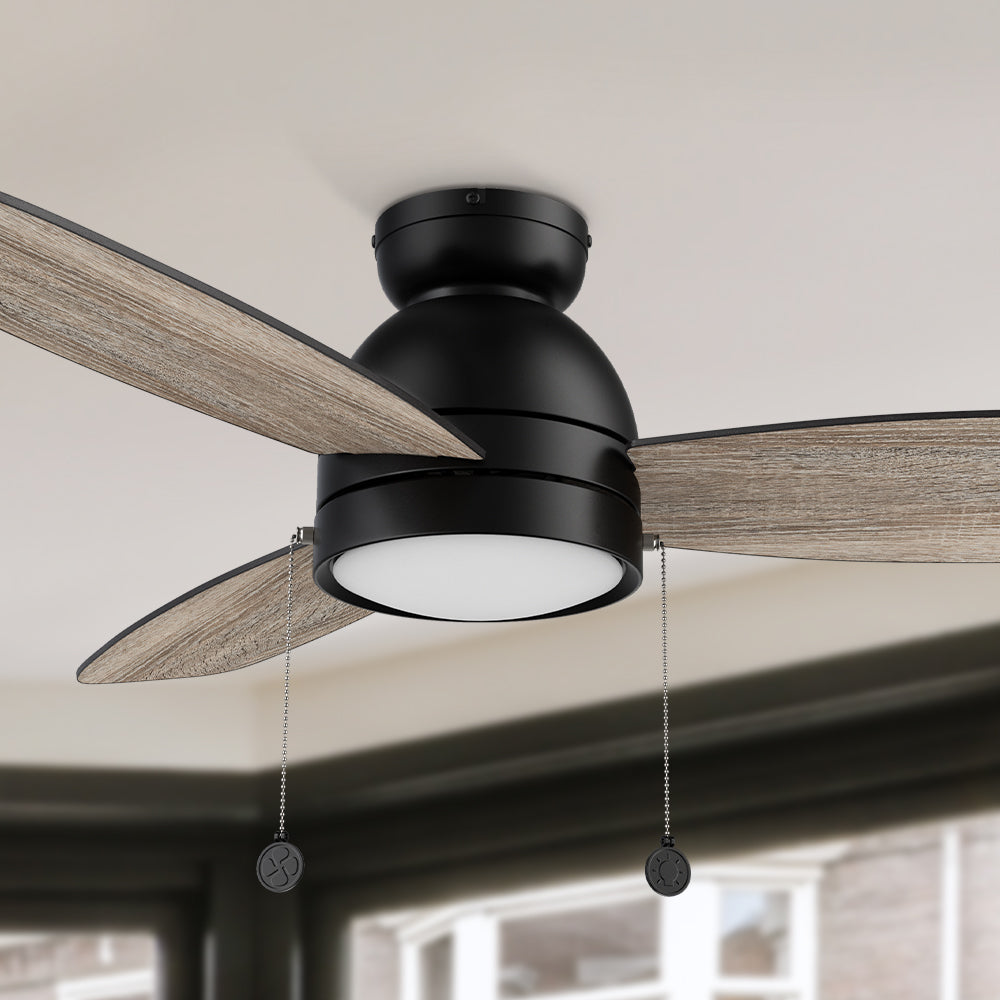The image showcases a modern, clinical-style ceiling fan prominently displayed as though for sale. The cream-colored ceiling is bordered on the back wall by a black wooden trim that delineates the space. The fan is centrally suspended from the ceiling and features a simple cylindrical black motor housing with three rounded, light wood-tone blades extending outward, though they are slightly cut off on the left and right edges of the frame. A downward-facing spotlight, which is part of the fan, emanates a flat, white light from its base. Two string pull-switches with icons for fan speed and light brightness dangle on either side. The background reveals the tops of a couple of windows with a small stretch of sheetrock wall above them, further leading visually to a view of another outdoor window from an adjacent property, indicating the space is indoors. The walls and ceiling share the same neutral, non-white color, adding to the clean, minimalist aesthetic of the scene.